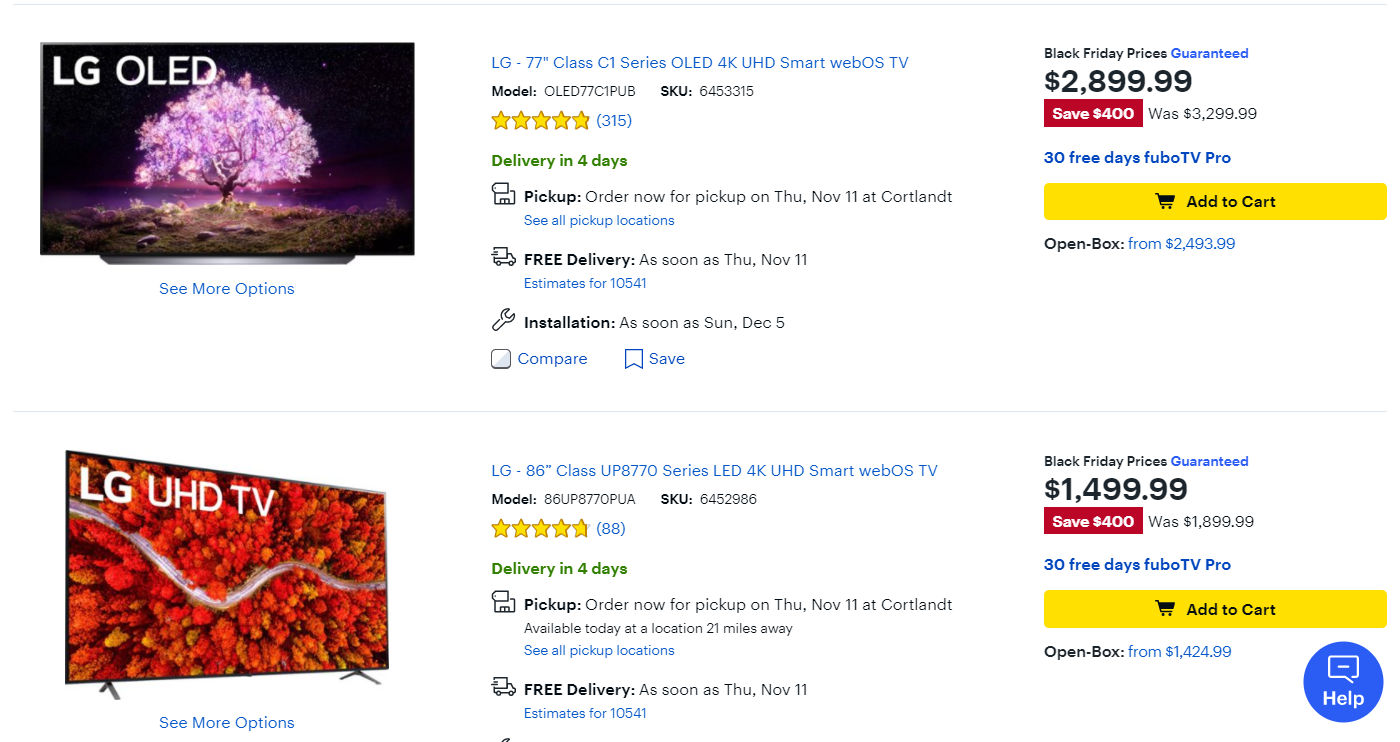Caption:

A detailed screenshot of a Best Buy desktop application showcasing their Black Friday deals. On the top left, there's an image of an LG OLED Smart TV. Below the image, a "See More Options" link is available. The background is predominantly white, with the centerpiece being the highlighted offer for an LG 77-inch Class C1 Series OLED 4K UHD Smart webOS TV. 

The product details include:
- Model: OLED77C1PUB
- SKU: 6453315
- Rated 5 stars by 315 reviewers
- Delivery available in 4 days

To the right of the TV image, a bold text proclaims "Black Friday Prices Guaranteed." This TV is priced at $2,899.99, marked down from its original price of $3,299.99—highlighted in red to emphasize a savings of $400. The purchase comes with 33 days of Fubo TV Pro subscription. A conspicuous yellow button with a cart icon offers an "Add to Cart" option. Additionally, there's an option to buy the TV as an open-box item starting at $2,493.99.

Below this feature, another LG UHD TV offer is showcased. This time, it's an 86-inch Class UP8770 Series LED 4K UHD Smart webOS TV priced at $1,499.99, down from $1,899.99, also offering a $400 saving.